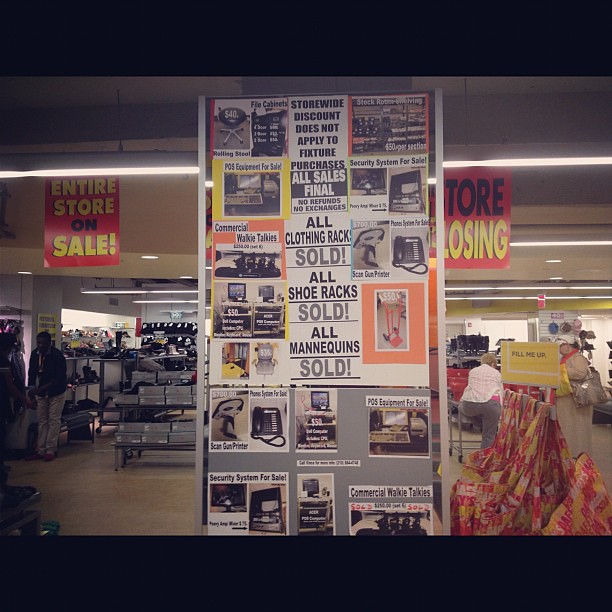This close-up photograph captures a detailed look inside a department store that's going out of business, prominently featuring a tall rectangular sign. The sign, central to the image, is plastered with a collage of posters and scattered pictures showcasing various products and sales information. From top to bottom, it displays messages such as "store wide discount does not apply to fixture purchases" and "all sales final, no refunds, no exchanges," emphasizing the finality of the clearance. Surrounding the sign are images of discounted items like a $40 swivel chair and other electronics. To the right of the sign stands a mannequin draped with a blanket and wearing a white hat. The store's tan floor and ceiling features banners declaring "entire store on sale" and "store closing," creating a vivid scene of a store in its final days, selling everything from clothing racks to electronics and fixtures.